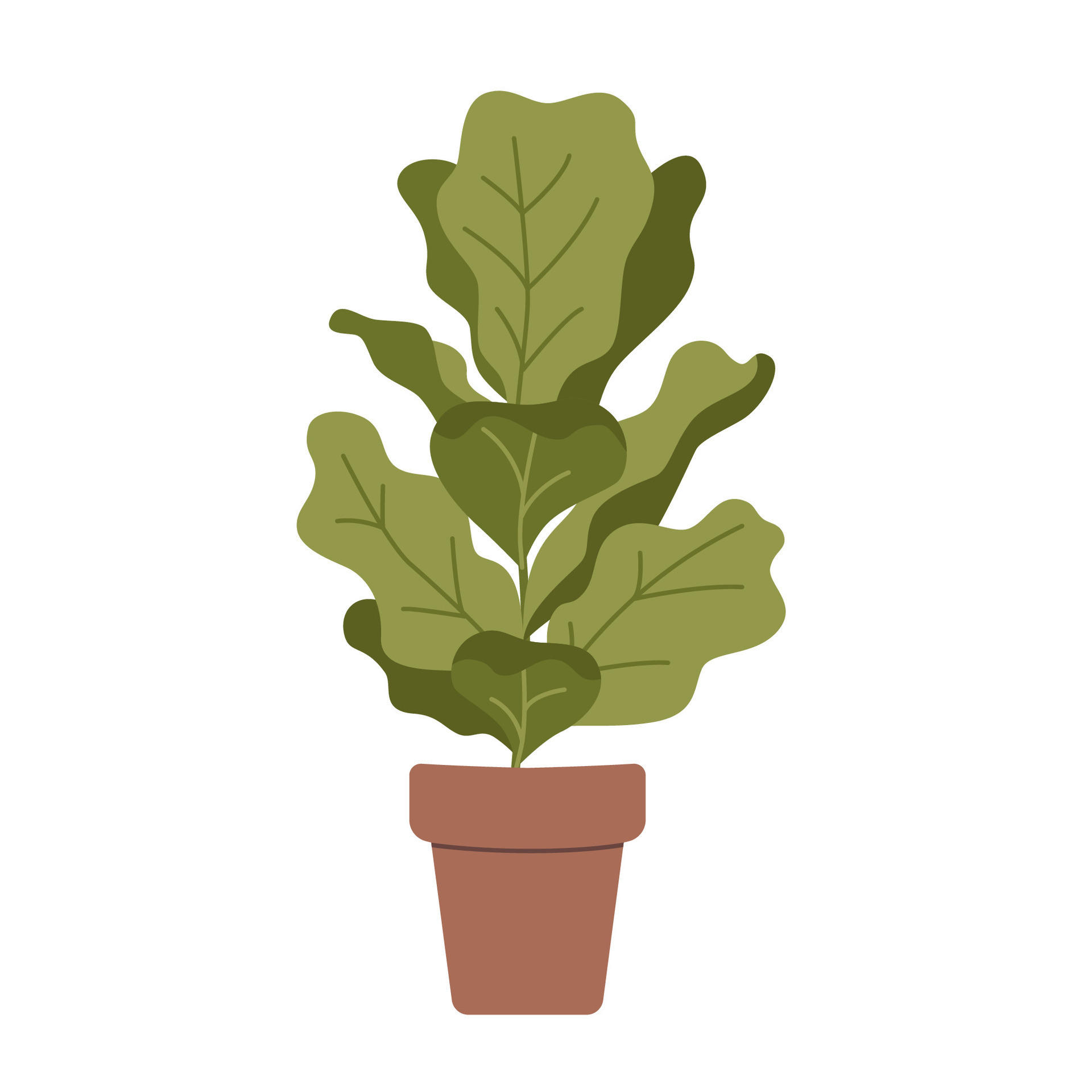This image features a computer-generated, cartoonish rendition of a potted plant centered on a plain white background. The pot at the bottom is a basic, squarish, reddish-brown or light brown color with a somewhat plastic appearance, although soil is not visible. Emerging from the pot is a plant characterized by large, squiggly leaves that range in color from light green to dark olive green. Each leaf has prominent veiny structures, with the vein colors contrasting based on the leaf's hue—dark veins on light leaves and light veins on dark leaves. The leaves are broad and number around ten, varying in their exact shades of green. Some subtle shadows from the leaves can be seen, enhancing the three-dimensional effect of this otherwise simplistic and stylistically drawn stock image.